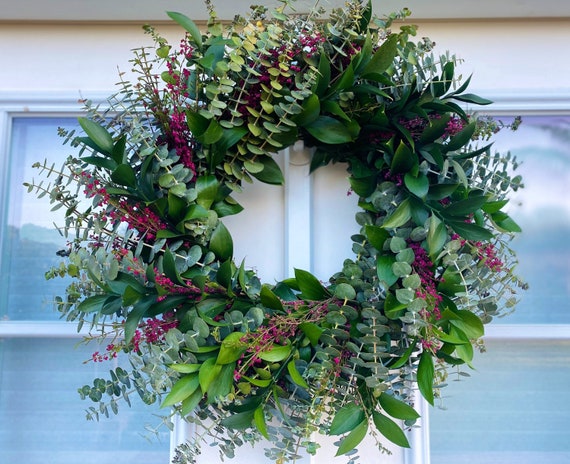This image captures a beautifully crafted wreath predominantly composed of lush, green eucalyptus stems. Adding a touch of color, the wreath features small accents of purple flowers interspersed throughout the arrangement. There are also subtle hints of white integrated into the design, further enhancing its visual appeal. The wreath is artistically hung on what appears to be a window-paned door or possibly a window, both characterized by a crisp white wooden frame. This natural and vibrant wreath stands out against the white backdrop, making it an enchanting and healthy-looking piece that draws the eye.